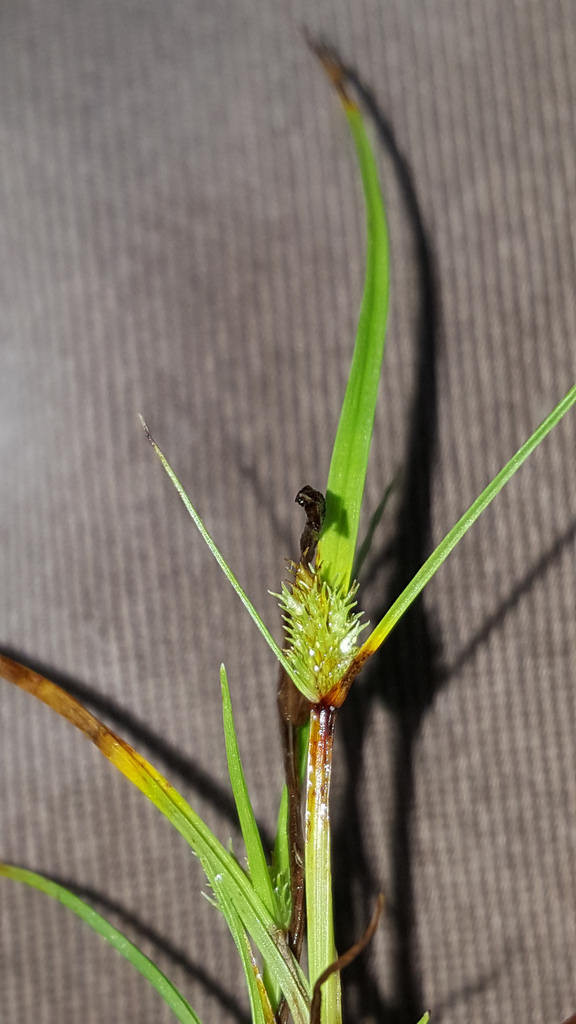The image depicts a close-up of a small, green plant with various shades of green and hints of brown and yellow on a few of its leaves, suggesting they may be dying due to nutrient absorption by the growing parts. The plant features thin, long, spiky leaves jutting out from its center, which houses a fuzzy bud with multiple protruding green elements. At the top of the bud, there is a black entity, possibly a caterpillar, insect, or even a piece of a dead leaf. The plant appears wet, indicating a damp environment or recent rainfall. The blurred gray background, resembling corduroy fabric, a couch, or pants, adds a contrasting backdrop that highlights the detailed and slightly prickly plant.